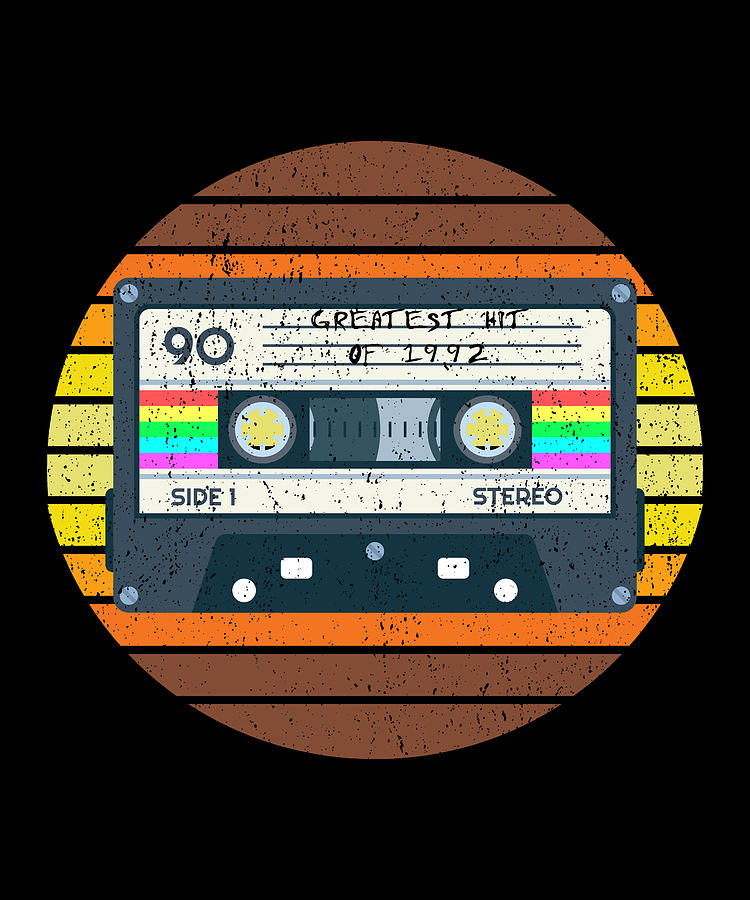This is a vintage-inspired graphic design featuring an artistic rendering of a cassette tape. The central element is a dark blue or purplish gray cassette tape with a white label inscribed with "Greatest Hits of 1992." The label also features the number 90 on the top left and the words "Side 1" and "Stereo" at the bottom left and bottom right, respectively. Additionally, there are colorful stripes in red, yellow, green, blue, and purple adorning either side of the cassette tape. The tape itself appears rewound, visible through the cassette’s transparent sections.

The background of the design is a black rectangular backdrop, on which a circular pattern composed of horizontal slits or striations lays beneath the cassette tape. These slits transition in color from brown at the top, to shades of orange and yellow, and back to brown at the bottom. The circle’s arrangement gives a segmented, almost wooden strip-like texture. The overall design is accentuated with black speckles, contributing to a grungy and rough aesthetic, enhancing the vintage vibe of the piece.